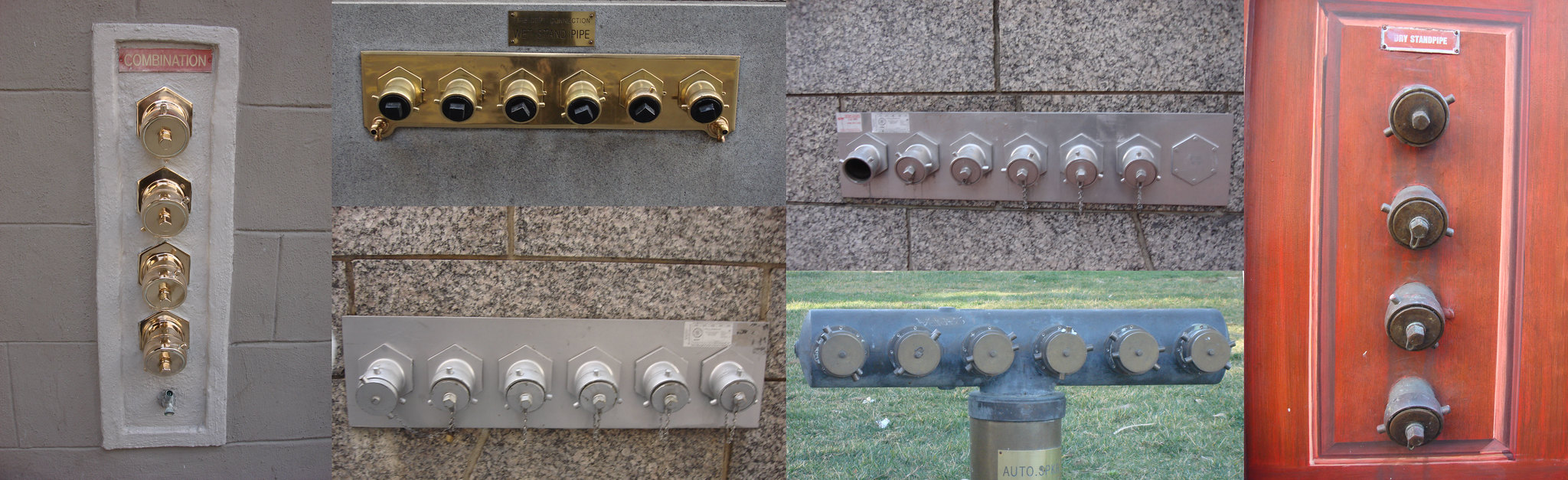The image consists of a long horizontal rectangular composition that integrates six separate photographs, each depicting a distinct device that seemingly involves cylindrical attachments or dials, potentially related to water systems or pressure controls. 

On the far left, there's a device mounted on a grey tiled wall, featuring four golden cylindrical dials on a metallic grey plaque, with 'Combination' written in white text on a red background at the top. Moving right, the next panel displays six gold dials with black edges, set against a gold background. Below this, there's another set of six dials, all silver and horizontally aligned, on a silver plaque. 

In the top right section of the middle series, another similar device features six silver dials with a noticeable hexagonal protrusion and a missing cap on the far end dial. Below this, there's a blue panel with grey dials attached to a silver post featuring a small plaque that reads 'Auto S' in black text. Finally, on the far right, there's a device on a red wooden background, likely a door, with four vertical bronze dials and unreadable white text on a red background at the top.